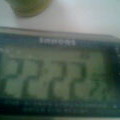This extremely blurry and poorly focused square photograph depicts a close-up of a digital alarm clock with an LED-style numeric display. The clock's surface is primarily a dull green color, showing the time as 22:22 with black digital numbers. The clock's frame is rectangular, featuring a brown top bordered by a blue plastic section beneath it. At the top center of this blue border, there are some silver-colored or white letters that are unclear due to the blurriness. The background is largely white, suggesting the clock is placed on a white counter or table, and there is an indistinguishable object nearby. The overall image quality makes it difficult to discern finer details.